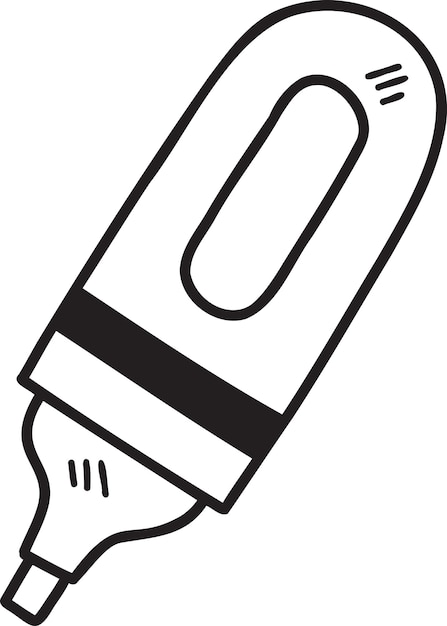This image is a clipart-style, black-and-white drawing of a marker with a transparent background. The marker has a thick black outline and a round body, with a broad oval-shaped window in the middle. Towards the end of the body, there is a long black rectangular stripe. The tip, which is thicker, emerges from a base at the end of the marker. The overall design resembles a cute, chibi-style anime drawing, featuring a simplistic and clean appearance, with no added fill colors. The top end of the marker is rounded, while the contrasting black and white elements highlight various structural details like the narrow neck leading up to the tip, similar to the opening of a glue bottle.